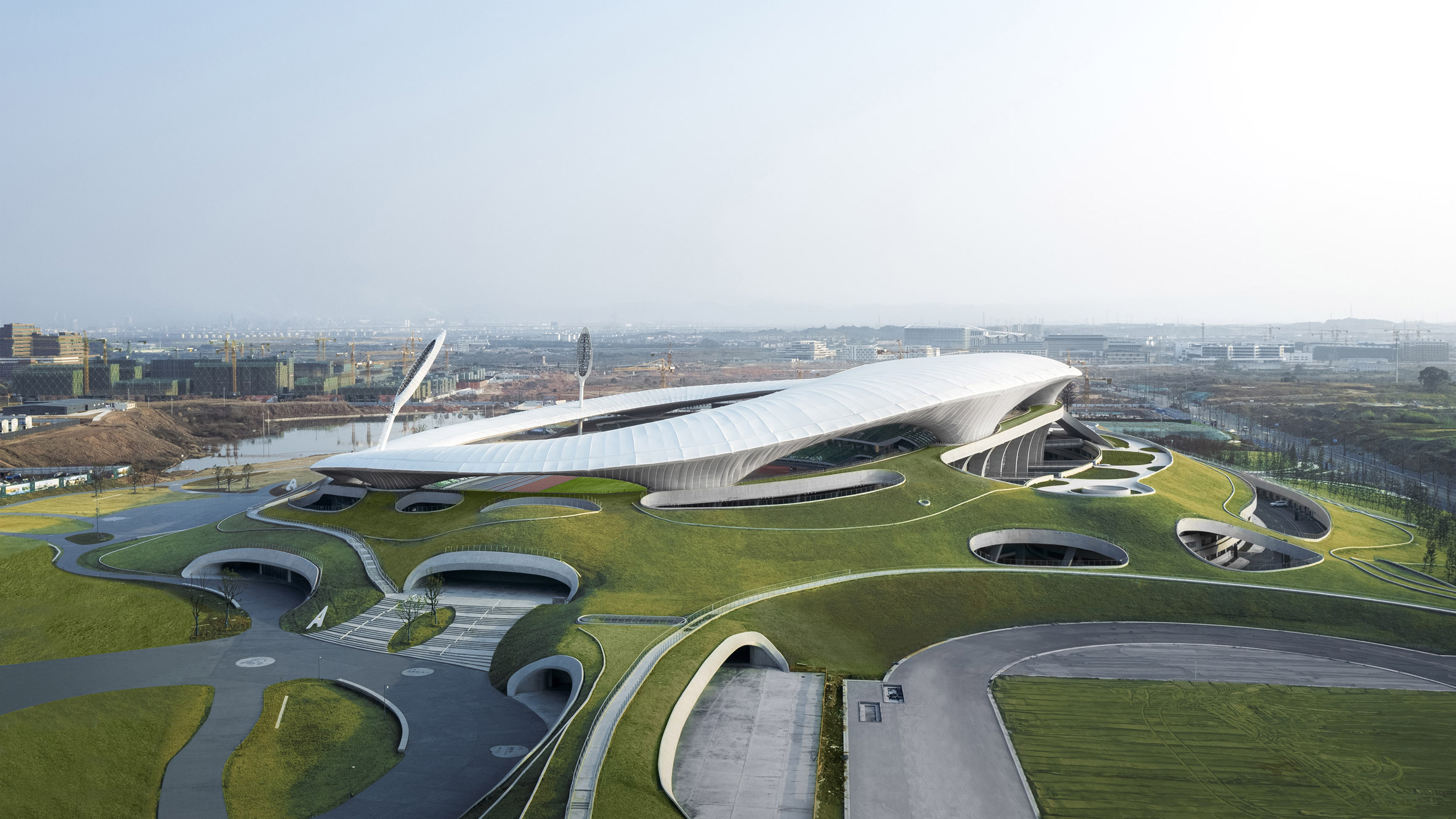From a slightly elevated viewpoint, perhaps from a drone or helicopter, the image showcases a peculiar stadium at its center, surrounded by a multi-layered parking structure that spirals around it. The stadium has an organic, wavy white ring with smooth columns and arches, giving it a sleek and surreal appearance. The surrounding landscape is a series of smooth, grassy hills cascading away from the stadium, dotted with roadways that lead to strange underground areas and tunnels. There are holes in the grassy terrain, seemingly to let light into subterranean spaces. On the left side, disproportionately large lights are visible along with a river. In the distance, an industrial-looking city shrouded in a smoggy haze completes the backdrop. The overall layout and elements, like nonsensical roadways and unrealistic features, suggest that this scene is a creation of AI, not a real place.